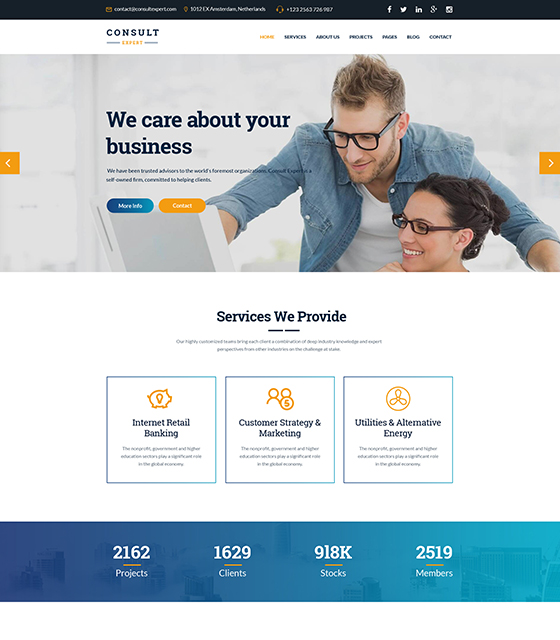The image appears to be a screenshot of a consulting firm's website. At the very top, there is a black banner featuring contact information and social media icons, including email, phone number, Facebook, Indeed, and Twitter. Below this, a white banner prominently displays the company’s logo, which reads "ConsultX," followed by a series of navigation options. The navigation menu includes the items: "Home" (highlighted in gold), "Services," "About Us," "Projects," "Pages," "Blog," and "Contact," all written in black.

Directly beneath the navigation bar is a rotating banner with images that can be navigated using gold arrows pointing left and right. Currently displayed is an image of a man and a woman, both wearing glasses. The woman is seated while the man stands beside her, leaning over to point at a screen they are both viewing with smiles. Captions below the image state "We care about your business," followed by two buttons: a blue one labeled "More Info" and a gold one labeled "Contact."

Further down, the section titled "Services We Provide" outlines various areas of expertise. This section includes three highlighted boxes: the first box covers "Internet Retail Banking," the second focuses on "Customer Strategy and Marketing," and the third discusses "Utilities and Alternative Energy." Each box contains additional detailed text that is too small to discern.

At the bottom of the webpage is a blue banner that summarizes some impressive statistics about the company: they have completed 2,162 projects, serve 1,629 clients, manage 918,000 stocks, and employ 2,519 members.